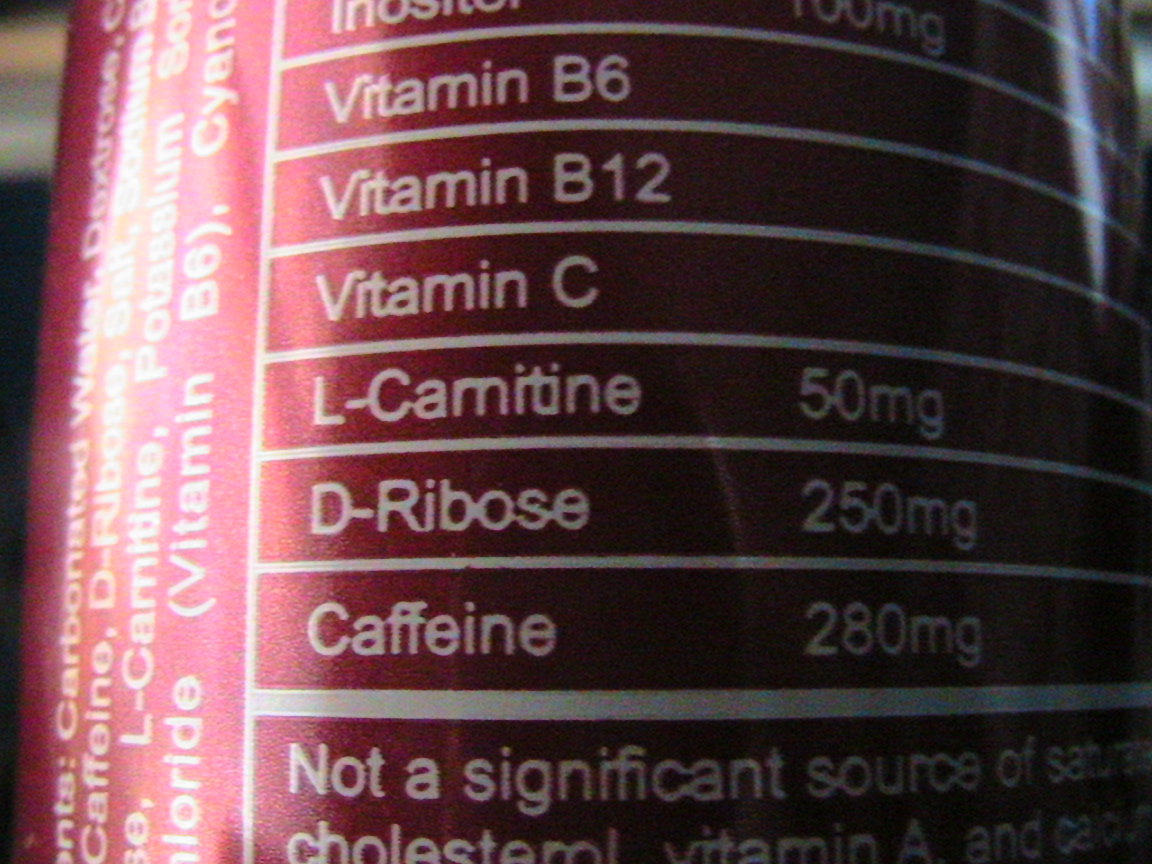The photo showcases a close-up of a nutrition label on a metallic, pinkish-red can, likely an energy drink. The can's surface features a shiny metallic paint, and the text on the label is printed in white, enhancing readability against the colorful backdrop. The image focuses on a breakdown of nutritional information, listing vitamin B6, vitamin B12, vitamin C, L-carnitine (50 mg), D-ribose (250 mg), caffeine (280 mg), with a note indicating it's not a significant source of saturated fat or cholesterol. The label also mentions vitamin A and contains a warning about the nutrient contents. On the left side of the label, oriented vertically and partially obscured by glare, the ingredients include carbonated water, caffeine, D-ribose, potassium, chloride, dextrose, and salt. Some portions of the text are cut off or illegible due to the zoom and glare, highlighting the curve of the can and making some words difficult to decipher clearly.